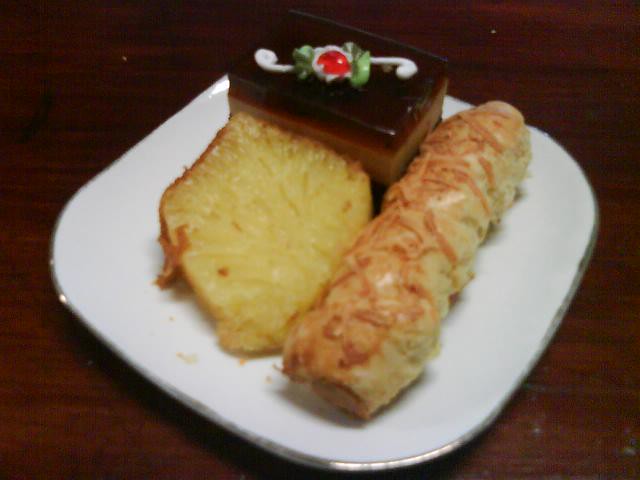The image showcases a white ceramic plate with a silver metallic outline, placed on a brown wooden table. The plate holds an assortment of pastries and desserts. Dominating the top left, there's a piece of cake resembling tiramisu with layers of light yellow filling and darker chocolate layers at the top and bottom. This piece is beautifully adorned with a red cherry on top, accompanied by a white decorative flourish and green embellishments, possibly floral designs. Below this, in the bottom left, is a rectangular pastry, possibly a hash brown or a pineapple-flavored dessert, displaying a distinct tan color with brownish crusty edges. Additionally, there's a long cylindrical pastry with a yellowish base and brown hues along the top, giving it a browned, crusted appearance. The picture suggests a nostalgic feel, reminiscent of the 80s or 90s.